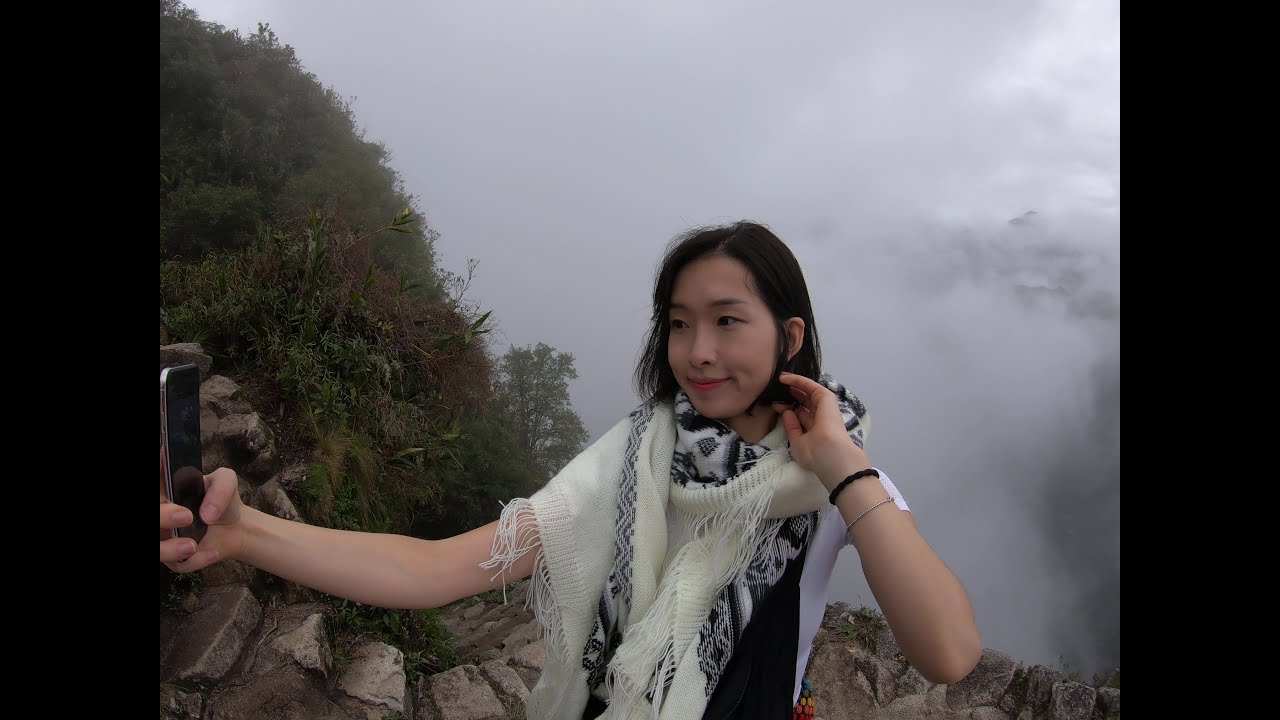In this square-shaped image, a young Asian woman is taking a selfie on what appears to be the edge of a cliff, evidenced by the sky visible both below and above her. The background shows a cloudy sky with predominantly gray and white clouds, suggesting a high elevation with a misty atmosphere. The woman, positioned centrally, is dressed in a white scarf and a black and white short sleeve top, giving her a modern, urban look. She has short straight black hair and is holding a cell phone in her right hand. Her left wrist is adorned with a bracelet. On the left side of the image, there's an ancient stone stairway that seems to lead higher up the rocky, scarcely vegetated mountain. To the right, the steep cliff accentuates the high altitude with misty clouds blending into the background. The entire setting, basked in natural daylight, includes various colors such as green, brown, gray, white, tan, black, pink, and red, contributing to a vivid outdoor scene.